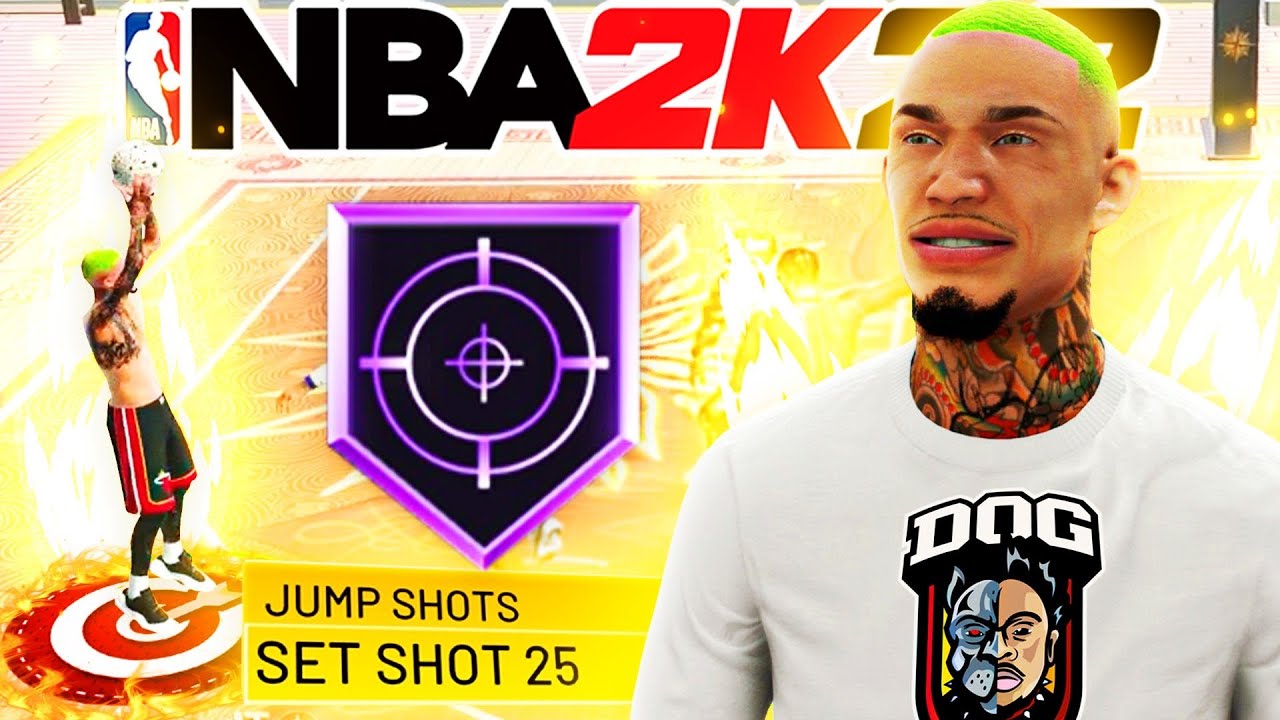The image is a horizontally rectangular screenshot from a basketball video game. At the top center of the frame, the NBA logo is displayed, followed by the text "NBA" in black and "2K" in red, symbolizing the popular NBA 2K series. 

On the right side of the frame, there is a detailed image of a player facing the upper left corner. The player is wearing a long-sleeve white t-shirt featuring a graphic of a dog and another image below it. The player's distinctive features include a large neck tattoo, a black goatee, and neon green very short hair.

To the left of this main image, a smaller inset shows what appears to be the same player, recognizable by the same neon green hair. In this inset, the player is shirtless and wearing shorts, captured in an action pose with a basketball held above their head.

Positioned between these two images, at the bottom of the frame, are the words "jump shot set shot 25," likely indicating a specific in-game move or setting related to the player's jump shot technique.